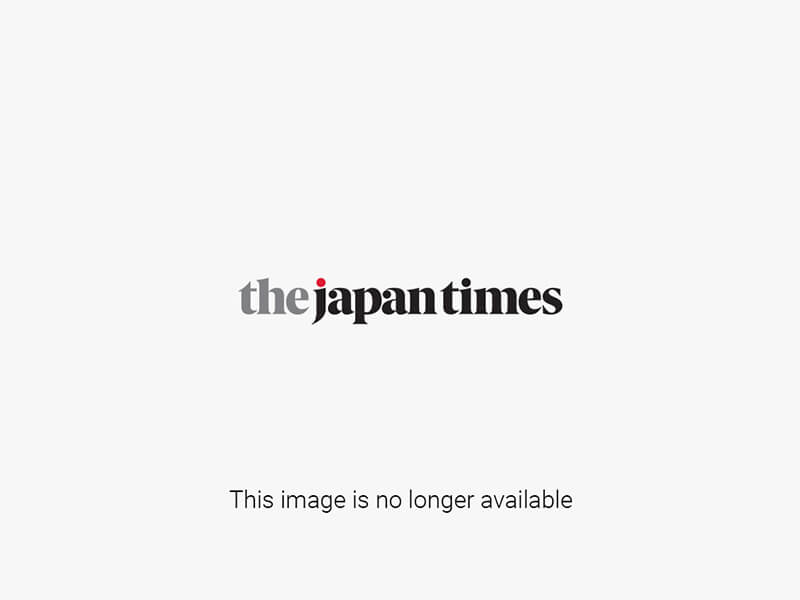This black-and-white photograph depicts a dramatic maritime scene with a city skyline, possibly New York City, shrouded in misty fog in the background. The skyline is characterized by numerous skyscrapers and high-rise buildings, with distant hills faintly visible. In the foreground, there are several boats crowded with people; the largest and closest boat prominently displays a Red Cross flag, indicating it might serve a medical or humanitarian mission. This boat is visibly overloaded with passengers, many of whom appear casually dressed, and features loose clothing and other items hanging from its sides. Additional boats, including smaller sailboats and possibly tugboats, are scattered in the mid-ground; some are also packed to their limits, suggesting a scene of mass migration or evacuation. The water appears gently undulating, adding to the overall impression of a tense yet orderly evacuation effort. The image has a vintage, worn feel, hinting at its historical significance, potentially relating to a period of significant migration or crisis.